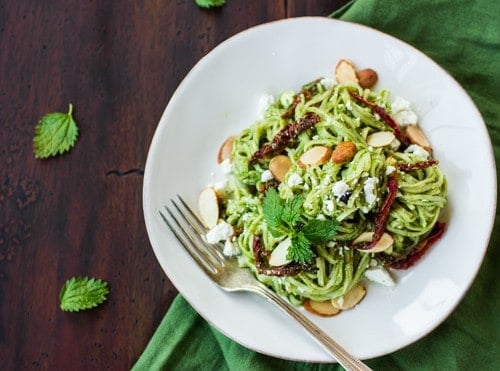A meticulously presented plate of green pasta, possibly pesto, sits on a clean white plate atop a dark wooden table partially covered by a green tablecloth. The pasta is adorned with slices of almonds, shavings of walnuts or pecans, and a generous sprinkling of Parmesan cheese, suggesting a rich, flavorful dish. The pasta appears to have a creamy sauce, ensuring it is not dry. Accompanying the pasta are garnishes of mint or parsley leaves and perhaps some slivers of mushrooms. A silver fork rests on the left side of the plate, and the entire setting is accentuated by the presence of loose mint leaves or similar greens scattered nearby, contributing to a fresh and appetizing presentation.